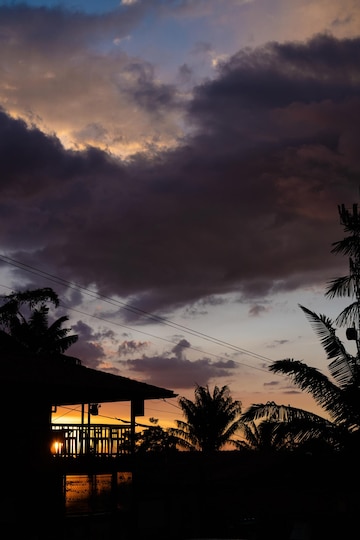This is a portrait-oriented photograph capturing a coastal scene at dusk, dominated by a dramatic, dark, and brooding sky filled with clouds, which occupies the top two-thirds of the image. The setting sun casts a reddish-orange glow behind a silhouetted house with a deck on the left-hand side of the lower third of the frame. Amid the shadows, only the black outline of the house, deck, and surrounding palm trees and foliage can be discerned. Just below the deck, a sliver of water is visible, reflecting the dim light of the disappearing sun. Power lines run diagonally above the house and trees, blending subtly into the darkening sky.